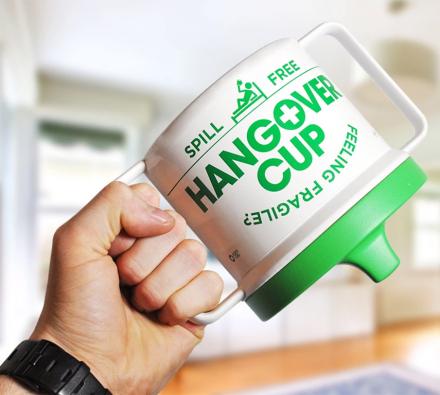In this image, a Caucasian man’s left hand, adorned with a black watch, firmly grips an unusually large, white cylindrical cup. This distinctive cup, designed as an adult sippy cup, stands out with its green top and green text that reads, "spill free hangover cup." Surrounding the text are the words "feeling fragile" wrapped around in green letters. Additionally, a stick figure cartoon is depicted drinking from the cup while lying on a bed, reinforcing its purpose for hangover recovery. The cup is equipped with two sizable, almost rectangular handles, allowing a secure grip, aimed at preventing spills even when turned upside down. The blurred background suggests a domestic setting with white walls, windows, wooden floors, and a rug, further emphasizing the focus on the cup itself.